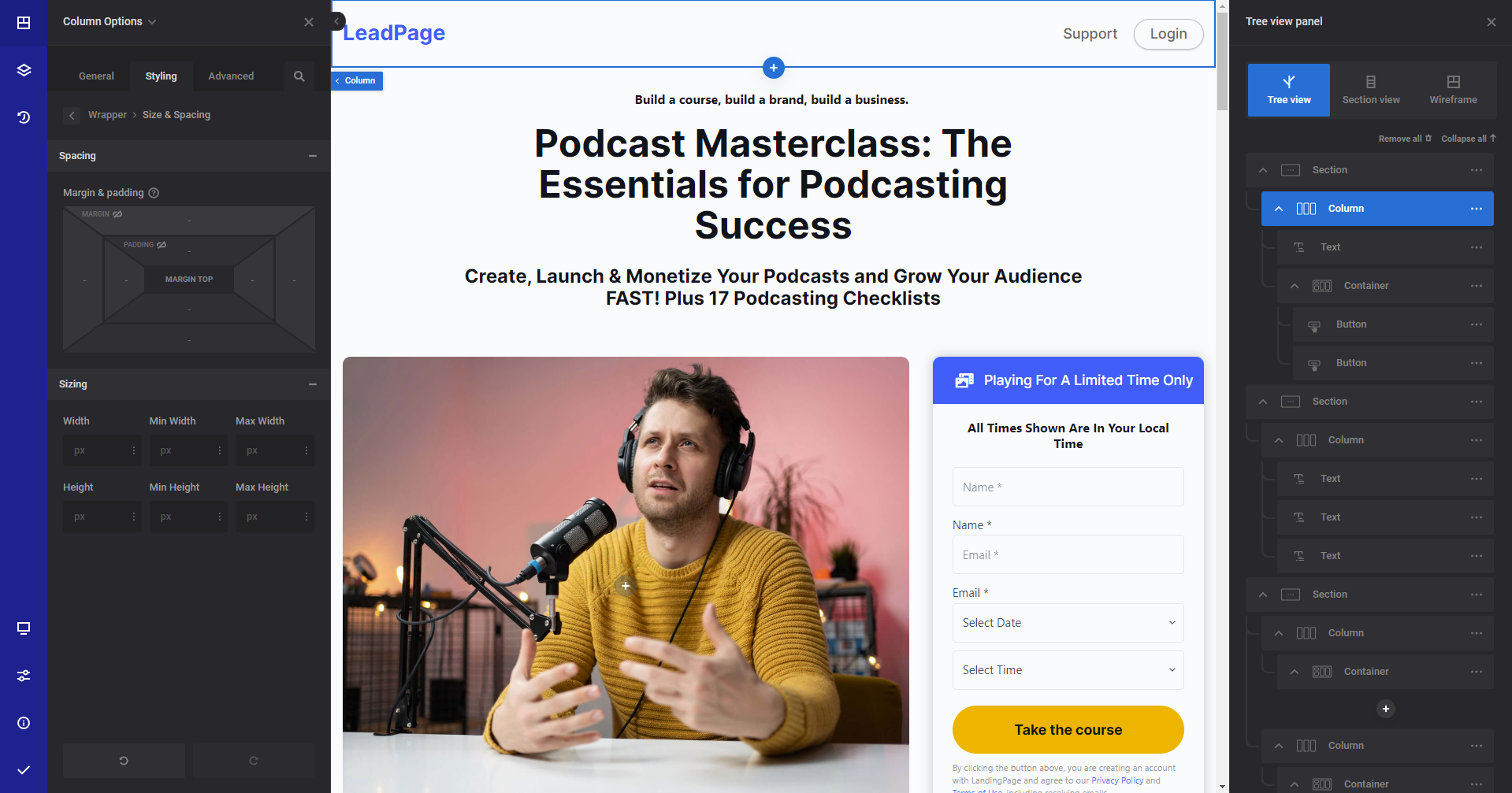In this image, the left side features a small blue box adorned with various icons including lines, a circle, and a square, along with additional icons towards the bottom. Adjacent to it is a larger black box with white text and several smaller black boxes inside.

Centrally positioned is a large white box outlined in blue, with a small black circle at the top and labeled "Lead Page." This box includes a "Support" label and a "Login" button. Below these elements is a tiny blue box with indiscernible text. A prominent circle with a plus sign inside contains the words "Build a Course, Build a Brand, Build a Business."

To the right, there is a vertical slider labeled "Podcast Master Class: The Essentials for Podcasting Success. Create, Launch, and Monetize Your Podcast and Grow Your Audience Fast. Plus 17 Podcasting Checklists." Next to this section is an image of a man speaking into a microphone, wearing headphones.

Below is a white box with a blue header, displaying small white envelope icons and the text "Paying for a Limited Time Only," and mentioning that "All times shown are in your local times." The box also includes fields for entering personal information such as name. A yellow box with the call-to-action "Take the Course" is visible.

On the far right, a black box contains a blue inset box, which mentions something related to time. Below this are several black boxes and a long blue box featuring colored elements and an upward arrow, along with a small white spot.